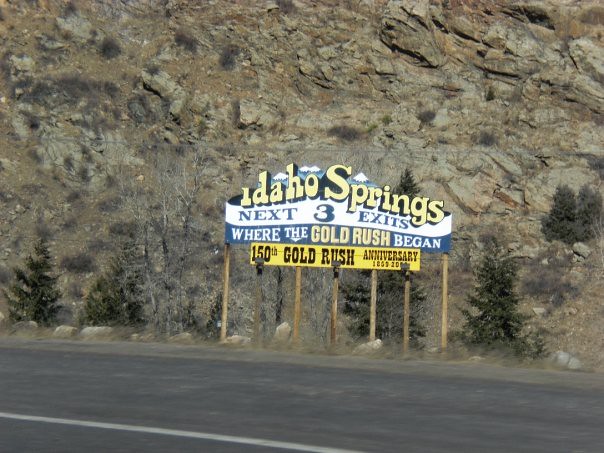The image depicts a stretch of dark gray paved road, marked by a solitary white line running along its length. Adjacent to the road, there's a scattering of tan-colored rocks that blend into the landscape, accompanied by patches of brown grass. The roadside scenery includes the tips of green evergreen trees, which gradually give way to a predominantly brown and tan hillside in the distance. Dominating the right side of the image is a series of tan-colored wooden fence posts that lead up to a prominent sign. The sign is adorned with white, blue, and yellow colors and reads: "Idaho Springs, Next 3 Exits, Where the Gold Rush Began, 150th Gold Rush Anniversary."